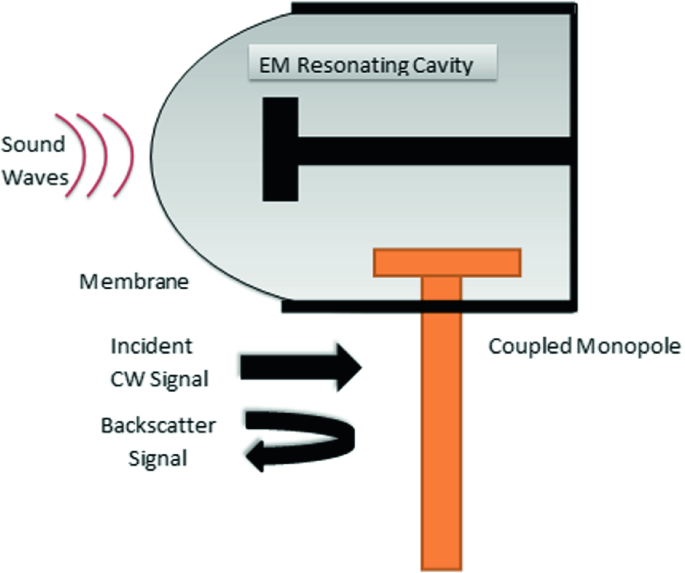The image appears to be a detailed scientific infographic, potentially from a textbook, illustrating the workings of an EM resonating cavity. At the top, bold black text against a light teal rectangle reads "EM Resonating Cavity." The central focus is on sound waves, depicted with a red semi-circle shape radiating from the waves. 

On the left side of the diagram, black text labels a sequence beginning with "Membrane," followed by "Incident CW Signal," an arrow pointing right, and loops down to "Backscatter Signal" with another curved arrow leading to "Signal." 

Additionally, there are notable geometric shapes included: a black rectangle, a smaller black rectangle to the side, and an orange T-shape composed of a vertical and a smaller horizontal rectangle labeled "Coupled Monopole."

Overall, the infographic likely aims to explain the interaction of sound waves within the EM resonating cavity, detailing how the incident and backscatter signals interact with the membrane and the coupled monopole structure.